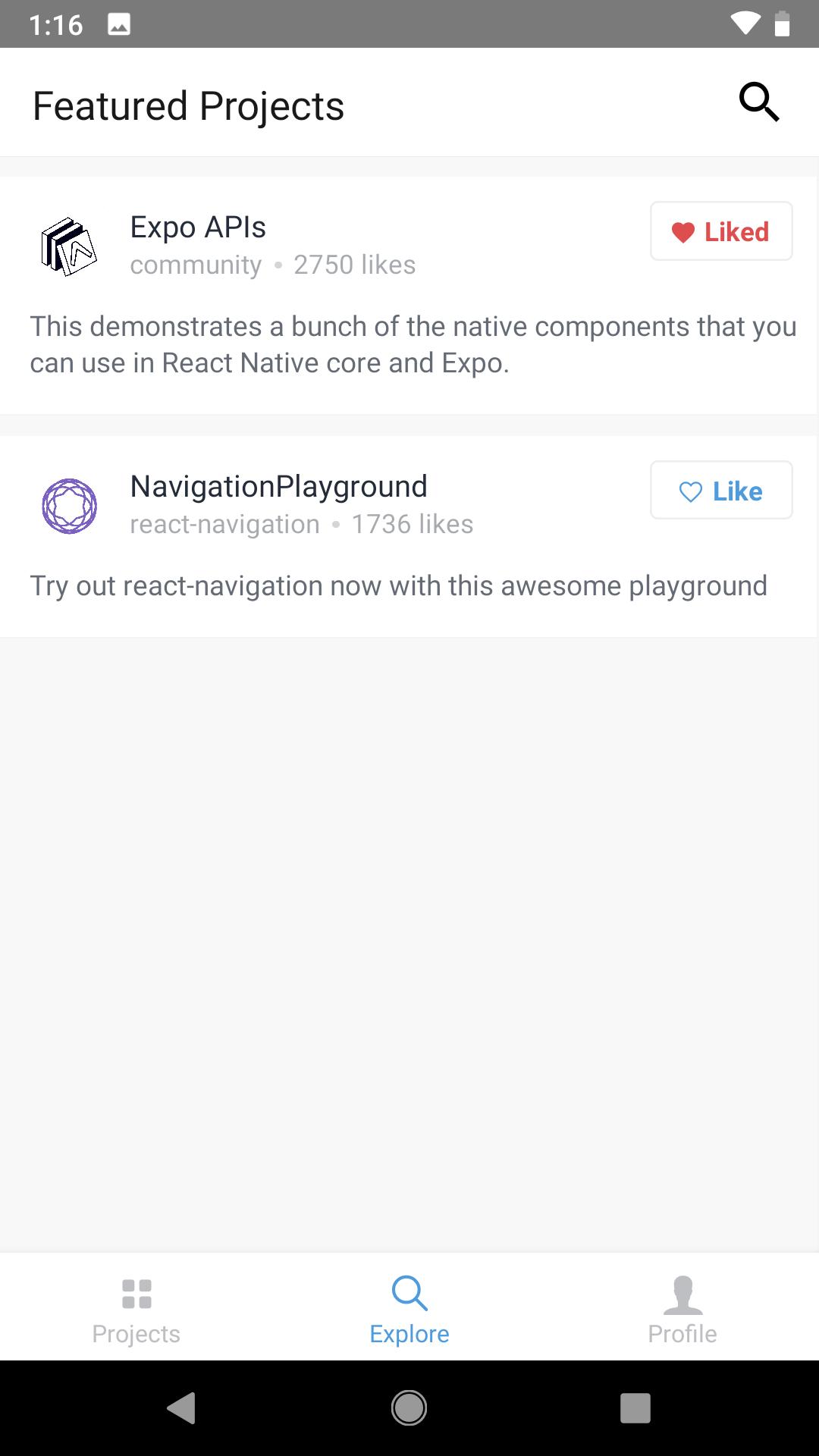The smartphone screenshot displays a detailed interface of an application with the top section of the device in grey. The status bar includes four icons: on the top left, the time (1:16) and a colored icon, while on the top right, there is a WiFi symbol and a page icon.

Beneath this grey section, the main content area has a white background. The black text header states "Featured Projects," listing two highlighted projects below.

1. **Expo APIs Community**  
   - **Likes:** 2,750  
   - **Like Button:** Positioned on the right, featuring a red heart icon.  
   - **Description:** "This demonstrates a bunch of the native components that you can use in React, Native Core, and Expo."

2. **Navigation Playground**  
   - **Likes:** 1,736  
   - **Like Button:** Positioned on the right, colored blue.  
   - **Description:** "Try out React Navigation now with this awesome playground."

At the bottom of the interface, there are three navigation buttons:
- **Explore:** Highlighted in blue. 
- **Project:** Grey. 
- **Profile:** Grey.

Additionally, the bottom-most section comprises the phone's system navigation buttons: Back, Home, and Recent.